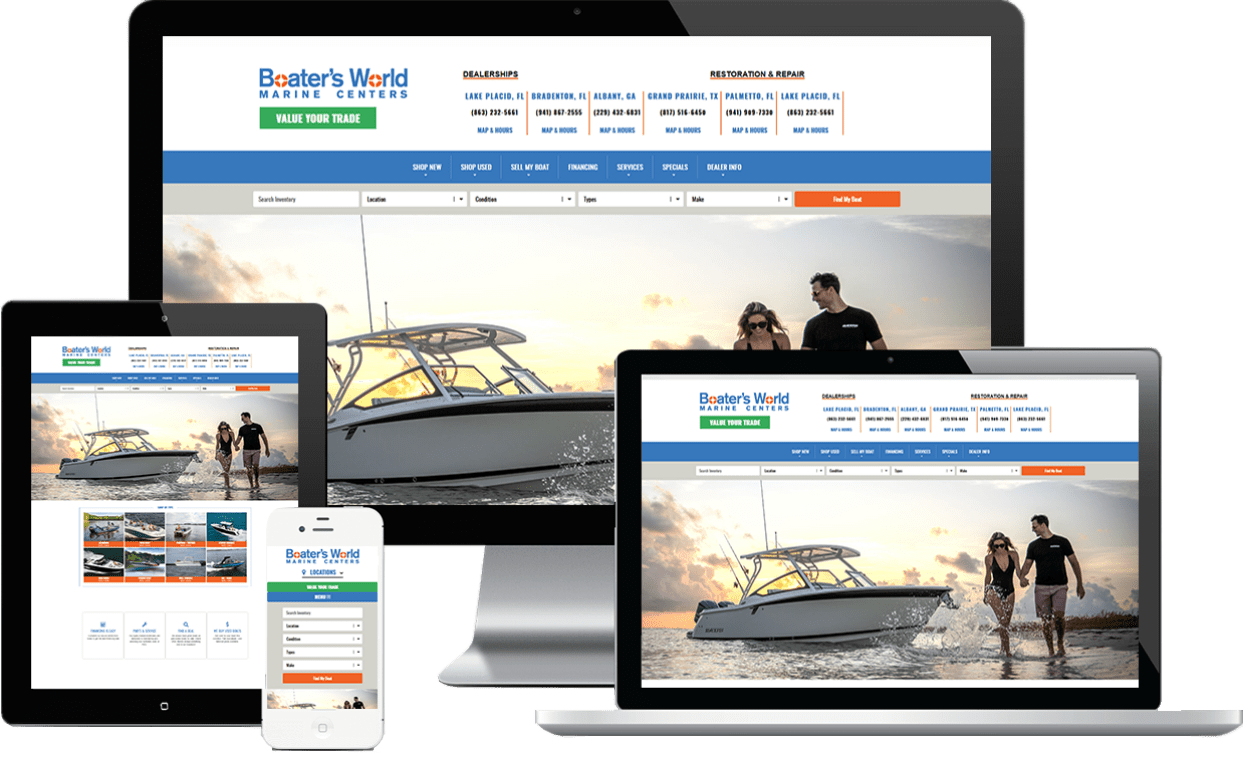The image is a screenshot displaying four Apple devices: a Mac computer, two iPads, and an iPhone. In the header of the screenshot, it reads "Voters World Marine Centers" in green, with the phrase "Value Your Trade" beneath it. At the top, partially legible text indicates something about a dealership and repair services. The central image features a man and woman walking hand-in-hand in the water, both smiling and dressed in swimwear—the woman in a black bathing suit, and the man in a black shirt and gray shorts. A beautiful sunset illuminates the scene, highlighting a large, white boat with black trim and silver accents next to the couple, capturing the water's splash as they wade. The screenshot demonstrates how users can log in or access various features across different Apple devices to find and customize their ideal boat, showing different categories based on user interests.